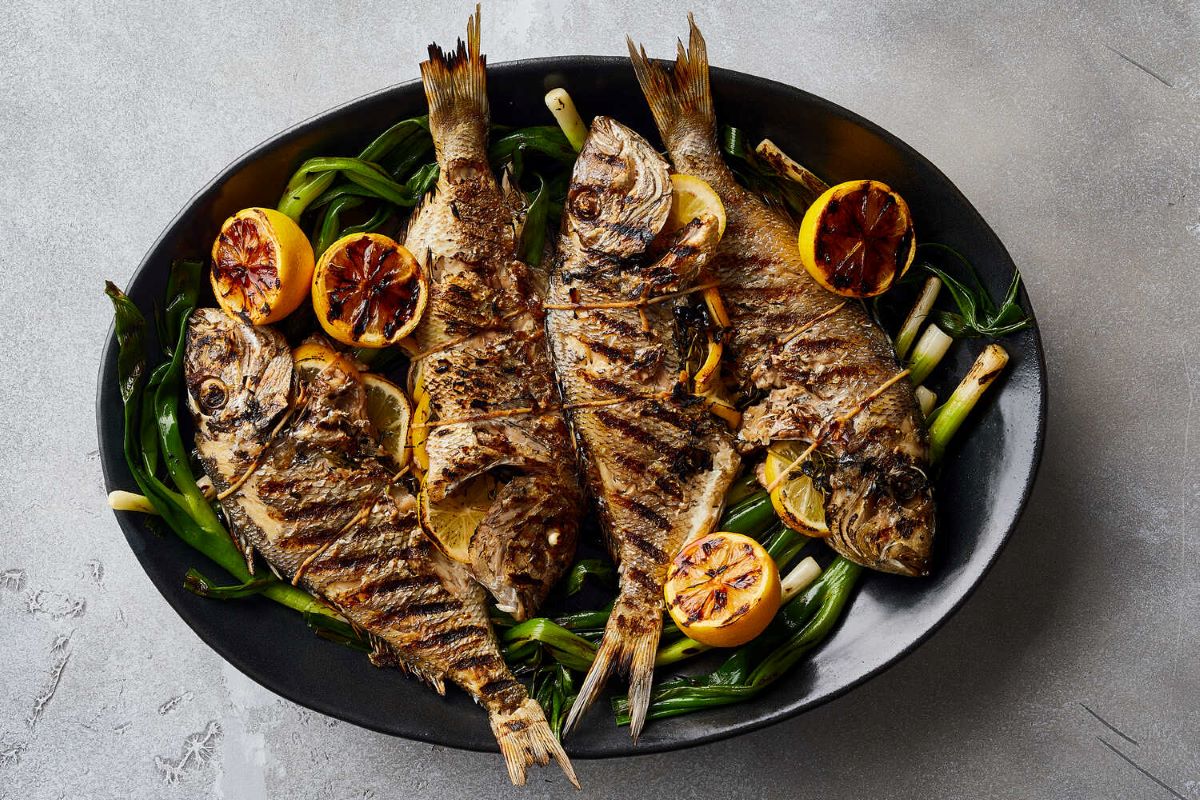In this image, a beautifully presented fish dish is displayed on a large, oval black plate, set on a dark gray surface, possibly a table or countertop with some scratches visible at the corners. The dish features four whole grilled fish, complete with heads, tails, scales, and skin intact, each bearing distinct grill marks. The fish are bound with twine and are carefully arranged on a bed of green onions. Accompanying the fish are several grilled lemon halves, both nestled around and stuffed inside the fish, enhancing the presentation and likely the flavor of the dish. Overall, the meal is presented family-style in a deep, slightly concave plate, making it an inviting and appetizing centerpiece.